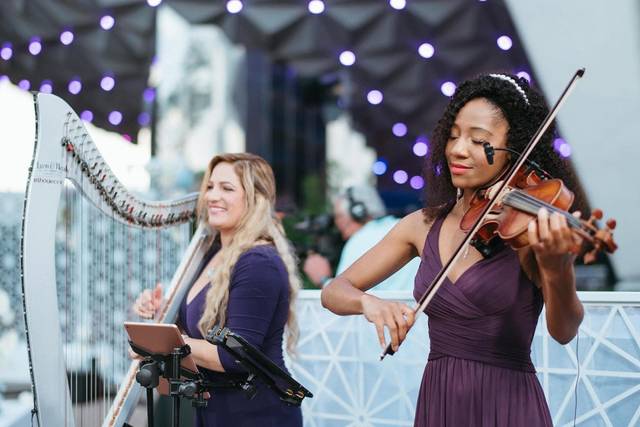The image captures a tender and evocative performance by two female musicians at what appears to be an outdoor event, possibly a wedding. The dark-skinned woman on the right, dressed in a plum-colored, wrap-style, sleeveless dress, is deeply engrossed in her violin playing, her eyes closed in a state of rapture. Her long hair is adorned with a headband, and a microphone is positioned over her violin to amplify her music. To her left, partially behind her, is a white woman with long, blonde hair cascading over her blue outfit. She is smiling warmly as she plays an elegant greenish, perhaps white, harp. Both musicians have music stands in front of them. The background is blurred but hints at festive decorations, including twinkling lights on a dark awning and possibly a screen with a snowflake pattern. The setting is likely a large room with partially visible people and a half-wall divider, contributing to the ambiance of this intimate and charming scene.